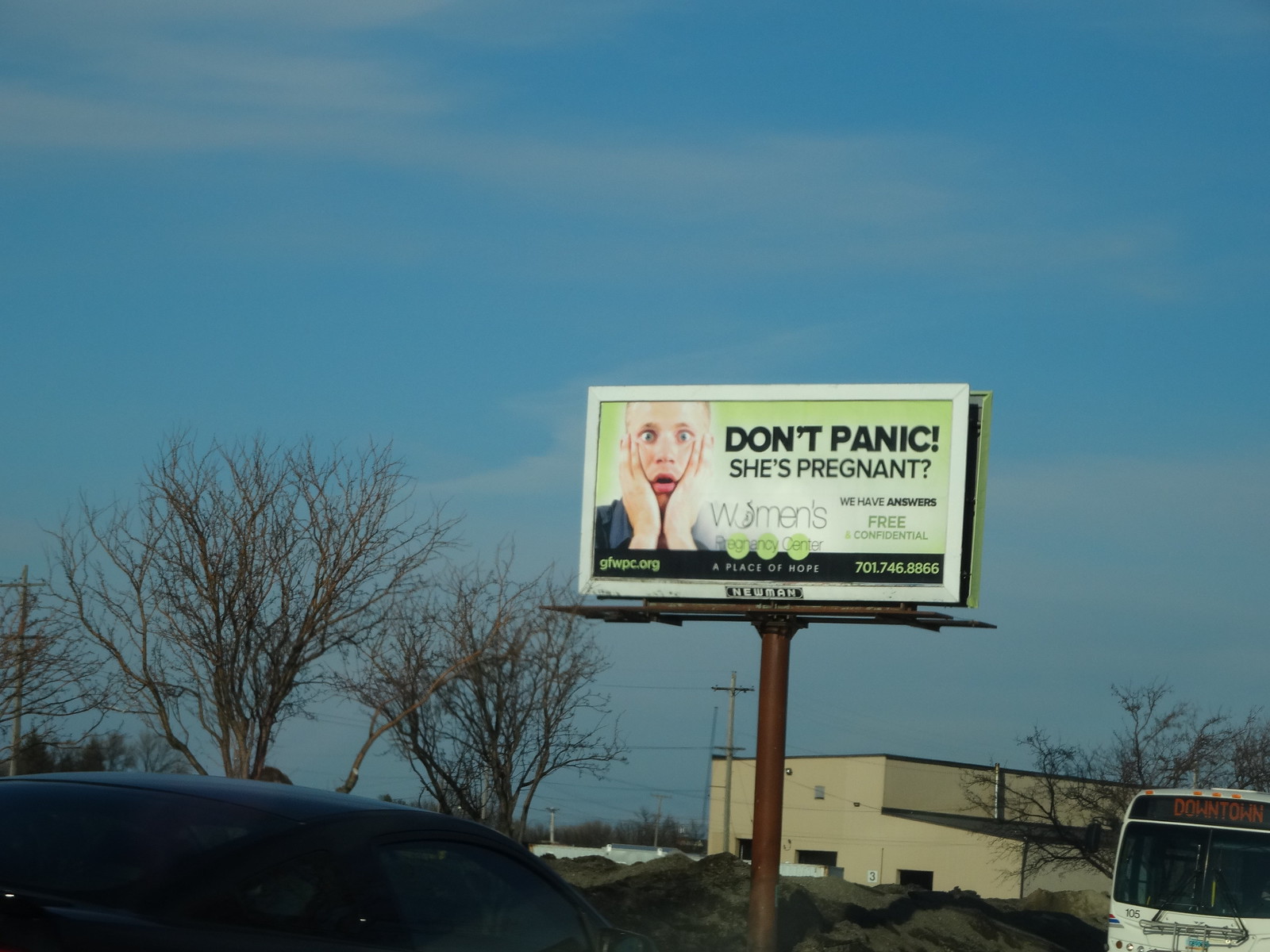The image captures a vibrant scene of a detailed billboard adjacent to a busy roadway under a striking blue sky with thin white clouds. The prominent billboard, mounted atop a tall brown pole, features a large, square design with a vivid green background. At the center left, a person with a surprised expression holds their hands to their face, staring wide-eyed into the camera with their mouth agape. To the right of this striking image, bold text exclaims, "Don't Panic, She's Pregnant!" Below this, additional text offers reassurance and support: "We have answers, free and confidential." The billboard is an advertisement for the Women's Pregnancy Center, branding itself as "A place of hope," and provides a contact number, 701-746-8866, as well as a web address, gfwpc.org. 

In the foreground, cars and a bus marked "Downtown" traverse the road, emphasizing the busy urban setting. The backdrop consists of a beige-colored building with a long, flat roof, likely a warehouse, and leafless trees suggesting a winter season. The overall scene is well set against the serene, yet vivid, blue sky scattered with a few wispy clouds.